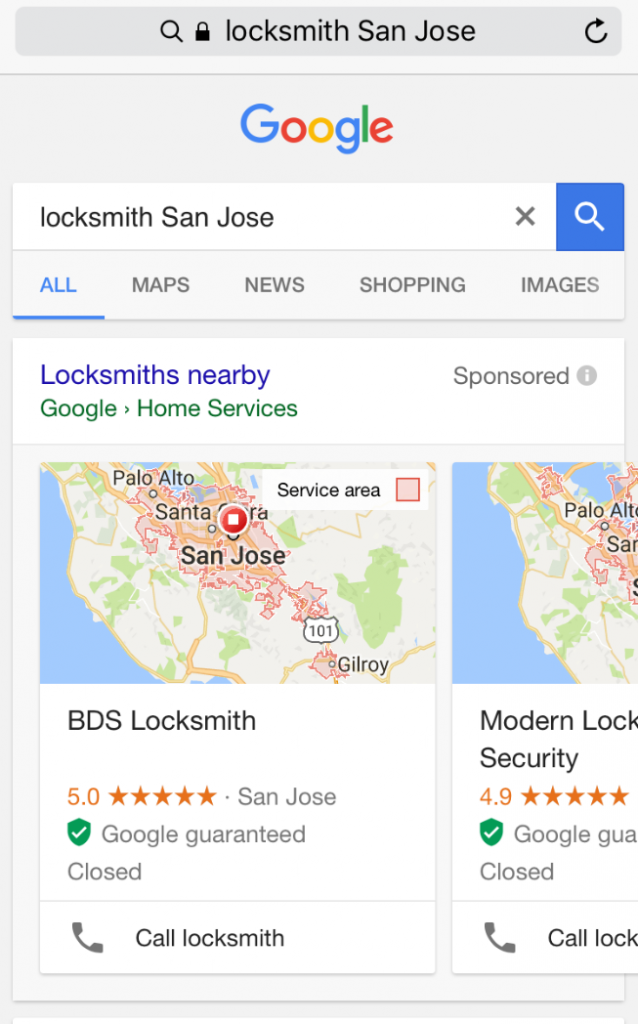The image depicts a Google search results page with a white background, featuring the search query "Locksmith San Jose" entered into the search box at the top. Below the search bar, the recognizable multicolored Google logo is prominently displayed, followed by a second search bar reiterating the query "Locksmith San Jose." Situated to the right of this bar is a blue button with a magnifying glass icon.

The navigation tabs below the search bar include "All," "Maps," "News," "Shopping," and "Images," with the "All" tab currently selected. The first search result appears below, titled "Locksmiths Nearby - Google Home Services," accompanied by a map of San Jose, California, highlighting a location marked with a red dot for BDS Locksmith. This locksmith has earned a 5 out of 5-star rating and is based in San Jose. Although displaying a Google Guaranteed seal, the business is marked as closed at this time. A phone icon beneath this listing offers the option to "Call Locksmith."

Adjacent to this listing is another partial map entry for "Modern Locksmith Security," also located in San Jose. This business boasts a 4.9 out of 5-star rating, alongside a Google Guaranteed seal, and is similarly noted as closed. A call button is similarly available beneath this listing for contacting the locksmith.